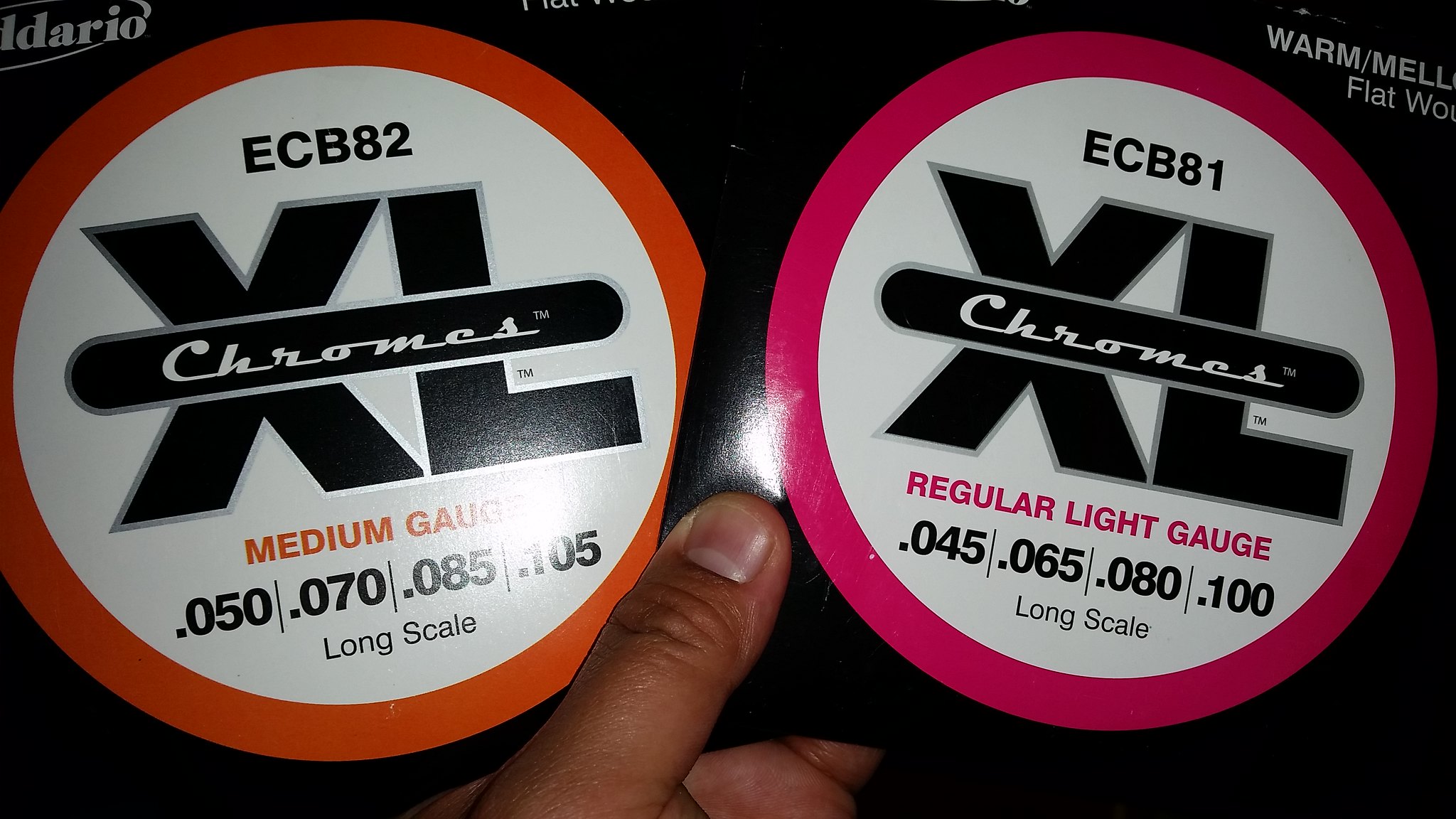The image is a close-up of someone's thumb holding two shiny labels against a black background. Both labels prominently feature the letters "XL" in large black font with the word "CHROMES" overlaid on top. The label on the left has an orange circular design and reads "ECB82 XL CHROMES MEDIUM GAUGE 0.050 0.070 0.085 0.105 LONG SCALE" in varying font sizes. The label on the right has a pink circular design and reads "ECB81 XL CHROMES REGULAR LIGHT GAUGE 0.045 0.065 0.080 0.100 LONG SCALE." These detailed and shiny labels highlight the specifications of the products, with distinctive color coding and clear text layout for easy identification.